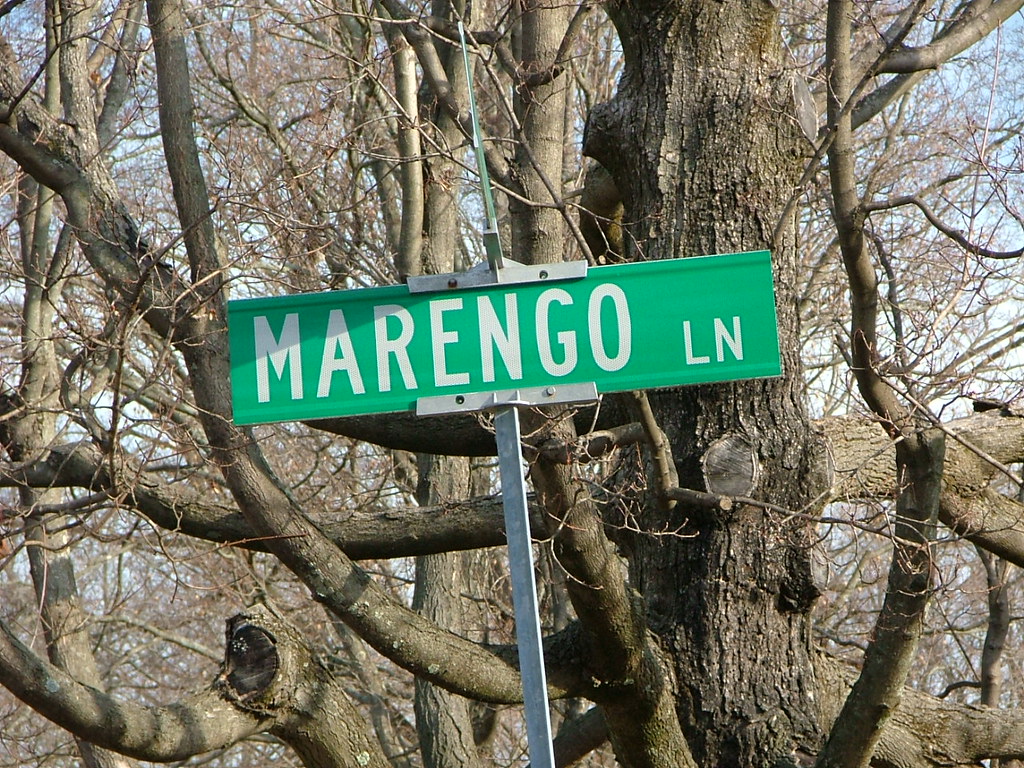The outdoor colour photograph prominently features a green North American-style street sign reading "Marengo LN" in off-white, light grey letters. The main word "Marengo" is in large letters extending across the vertical length of the sign's face, with "LN" positioned in smaller capital letters towards the bottom right corner. The sign is a slim, sleek, and narrow metal rectangle, slightly corrugated along its edges, mounted on a steel pole. Another sign is situated on top, facing away from the camera, making its text unreadable. Dominating the background is a large mature tree with a thick trunk and numerous branches, some of which are cut, extending in various directions. The branches twist toward the camera, upward, and to the sides, with a few other trees visible behind, all devoid of leaves. Small patches of blue sky and greyish white clouds peek through the dense network of branches. The predominant colors in the image are various shades of green from the sign, brown from the tree trunks, white from the text, and touches of blue from the sky, giving the scene a natural yet slightly stark winter feel.